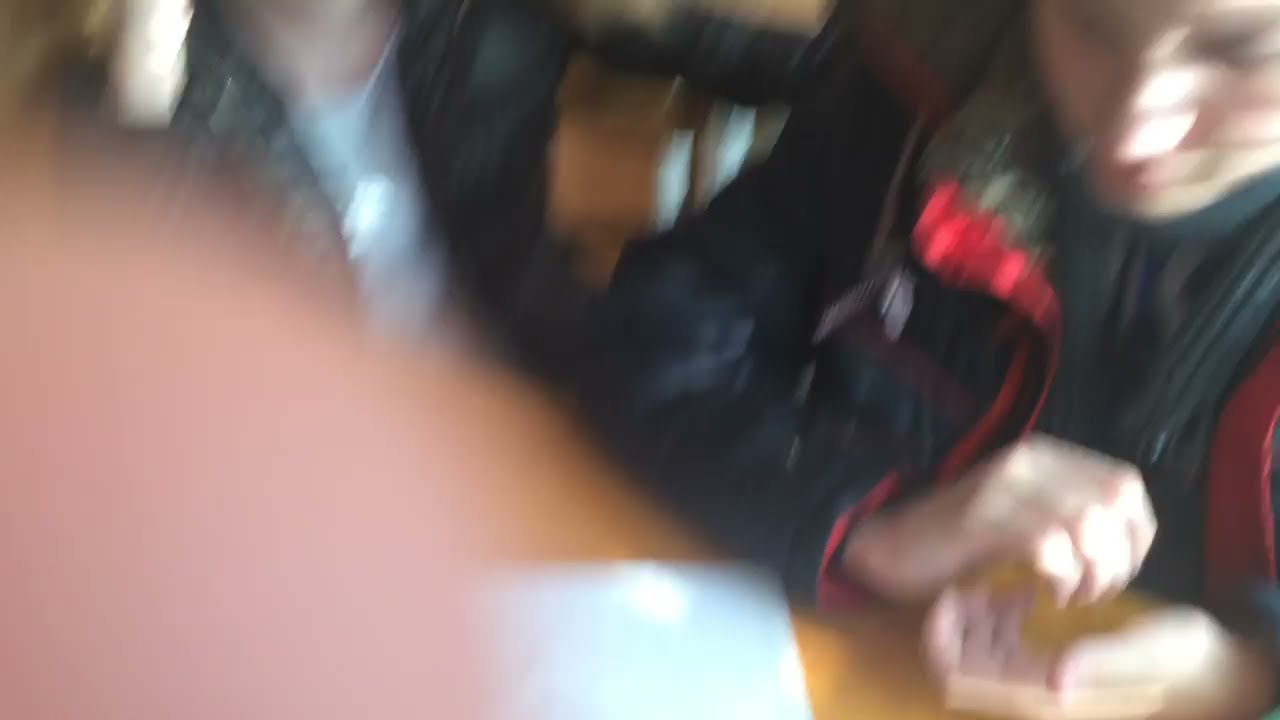In this blurry, out-of-focus photograph, a thumb or a beige spot obscures almost half of the image, particularly on the left-hand side, causing the photo to appear uneven and low quality. The scene depicts two individuals sitting at a desk or table indoors, possibly at a school. The central table holds a white rectangular sheet of paper. The person on the left, partially obscured, wears a dark jacket over a light shirt, while the person on the right is more visible, clad in a black and red jacket over green clothing and sitting with clasped hands, looking downward. The background features a young woman and a hint of a yellow square with some light and dark contrasting colors. The overall color palette includes tan, white, light brown, black, red, gray, and green.